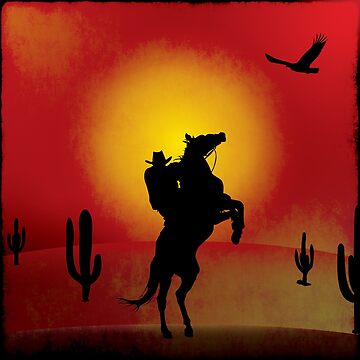The image is a striking silhouette drawing of a cowboy riding a rearing horse against a dramatic sunset backdrop. The cowboy, identifiable by his wide-brimmed hat, holds the reins tightly as the horse, standing on its hind legs with its front legs curled and head lifted towards the sky, captures a moment of intense action. The scene is set against a dark amber-red sky, with a large, muted yellow sun setting centrally. Silhouetted cacti populate the landscape, adding to the desert atmosphere, and the ground beneath the figures curves slightly, suggesting a hill or dune. Completing the composition, a solitary eagle soars in the upper right corner, adding a sense of wild freedom to the artwork. The primary colors used are varying shades of red, black, and yellow, enhancing the dramatic and rugged feel of the western scene.